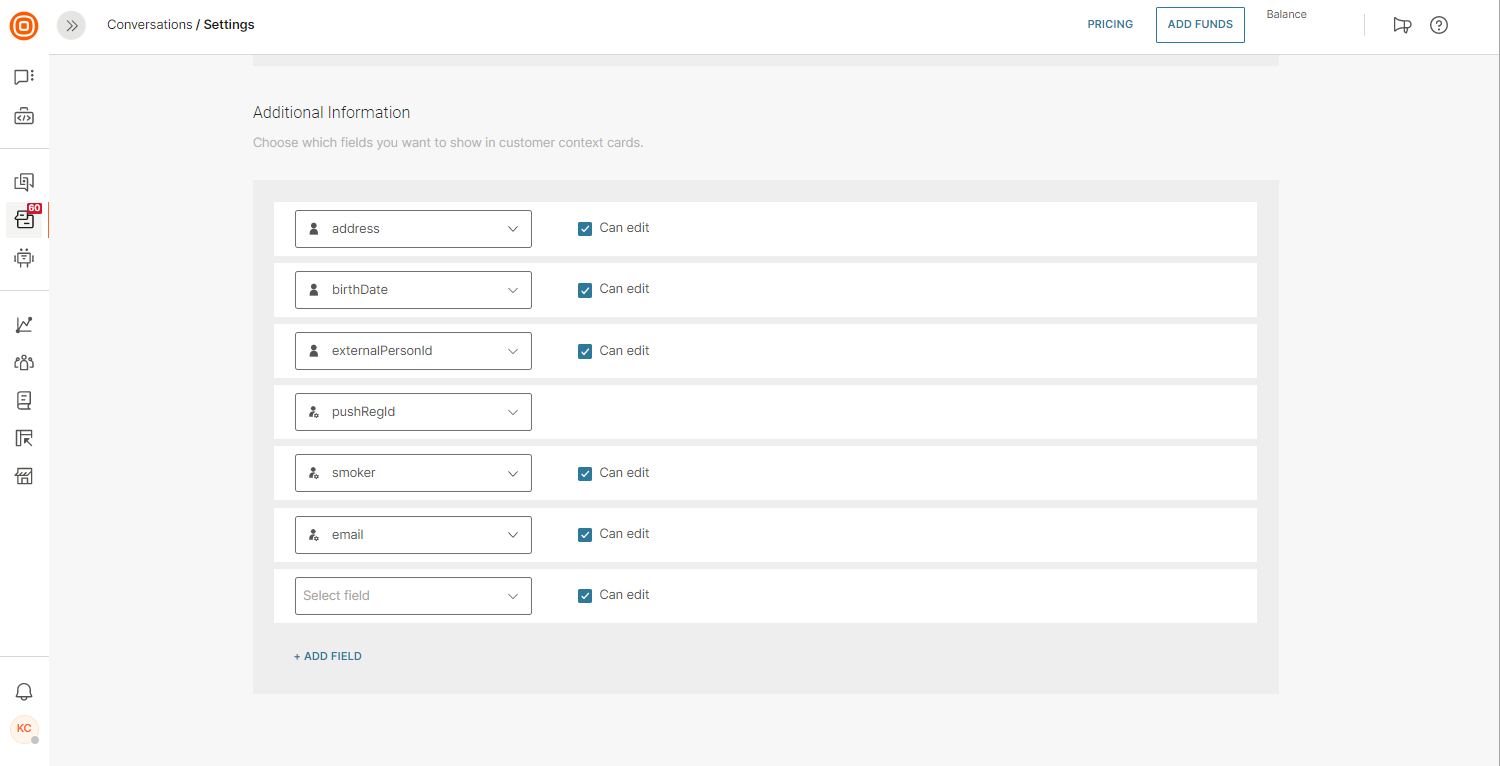The image displays a web page or settings interface set against a light gray background. 

### Header Area
- **Top Left**: An orange circle containing two small white squares.
- **Right of the Circle**: A double right arrow icon followed by the text "Conversations / Settings."
- **Further Right**: 
  - In blue text: "Pricing."
  - An "Add Funds" button next to a rectangular box labeled "Balance," which is in gray.
  - A megaphone icon.
  - A question mark icon.

### Sidebar
- **Left Vertical Sidebar**: Contains 12 icons, each representing different options.
- **Below the Icons**: The text "KC" in orange, accompanied by a light-orange circle.

### Main Section
- **Upper Left**: The text "Additional Information."
- **Instructions**: "Choose which fields you want to show in customer context cards."
- **Dropdown Fields**: A series of dropdown menus labeled as follows:
  - Address
  - Birthdate
  - Extreme
  - Person ID
  - Push Reg ID
  - Smoker
  - Email
  - An additional, unselected option labeled "Select field."
  - Below the dropdowns, in blue, it says "+ Add Field."

### Edit Options
- **Right of the Dropdowns**: Six options, each with a blue box containing a white check mark, indicating "Can edit."

This detailed description offers an intricate look into the components and layout of the web page or settings interface displayed in the image.